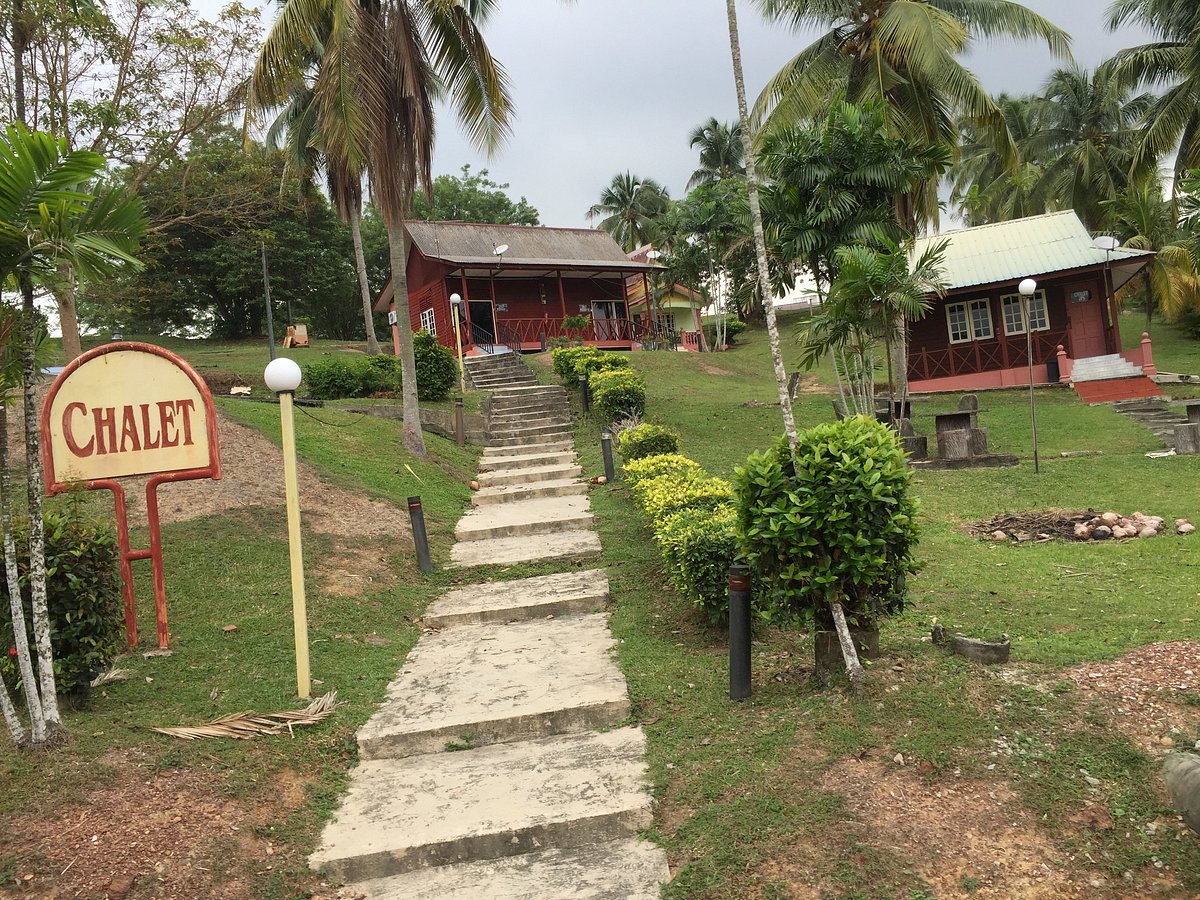The image depicts an outdoor scene in a tropical area featuring a set of concrete steps leading to two small, burgundy buildings reminiscent of bungalows or chalets. Palm trees and various bushes line the walkway on either side, while several rods that likely serve as lights stand along the path, though they remain unlit in the daytime. The building on the left has a medium gray roof, whereas the building on the right, which is slightly smaller, sports a white roof. A bright yellow sign with red writing, held by a red signpost to the left of the steps, prominently displays the word "CHALET." Additionally, regular trees are visible in the background, further enhancing the lush, tropical ambiance. The overall setting suggests a secluded, peaceful retreat such as a motel or a series of holiday bungalows, surrounded by greenery and equipped with outdoor seating areas for relaxation.